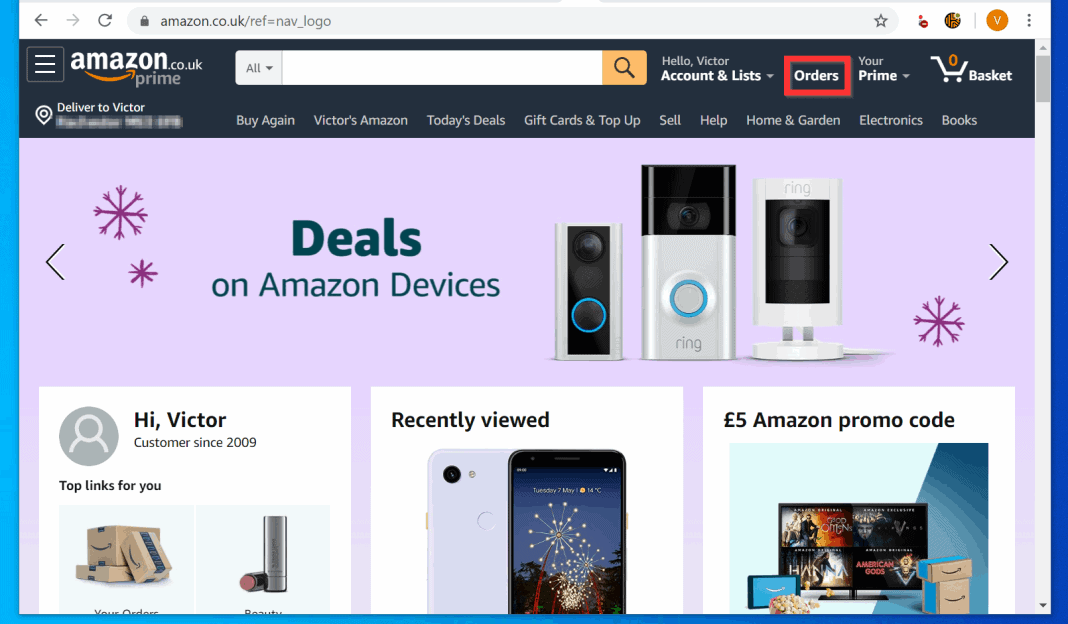The image captures a screenshot from the Amazon.co.uk website. In the upper left corner, the Amazon.co.uk logo is clearly visible, with the word "Prime" displayed just below it. The page greets the user by name, saying "Hello, Victor," near the top where account-related options such as "Accounts & Lists" are located. There is a red rectangle highlighting the "Orders" section, suggesting an instructional purpose to draw attention to that area.

Further down the page, a banner promotes "Deals on Amazon devices." Below this banner, the site acknowledges Victor as a customer since 2009. The "Recently Viewed" section features two cell phones, indicating Victor's recent browsing activity. In the lower right corner of the image, there is a £5 Amazon promo code displayed prominently. Personal information about Victor has been blurred out for privacy.